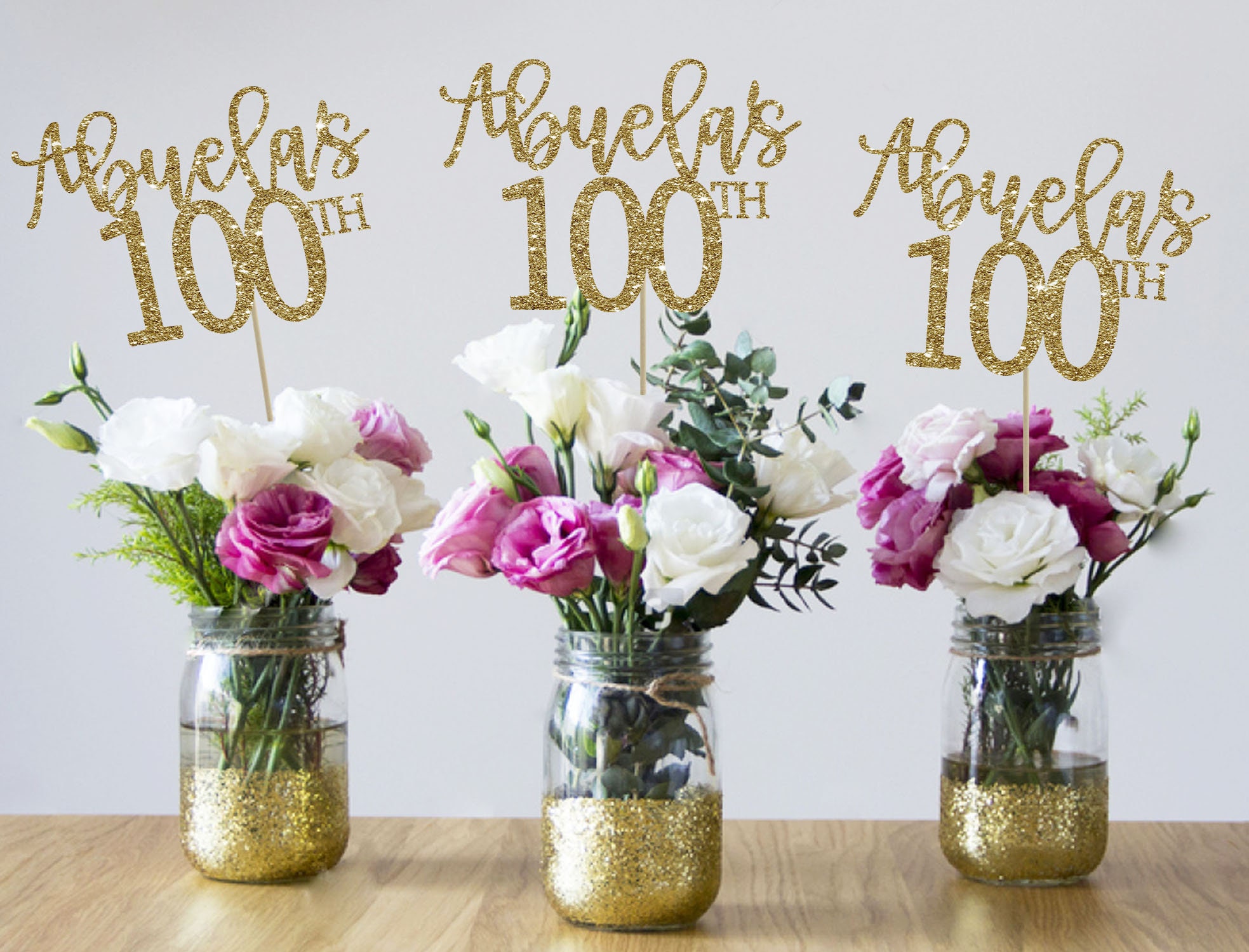The image showcases three round mason jars arranged on a medium brown, wood-grained table. Each jar is filled with water and has gold glitter settled at the bottom. Inside each jar is a lush bouquet featuring white and pink flowers, including carnations, white roses, and some green foliage, with the greenery varying between being more fern-like on the sides and resembling rose leaves in the middle. In addition, there are gold-colored sticks in the bouquets. Above the jars, a gold hand-lettered sign reads "Abuela's 100th," marking this as a celebratory decoration, possibly for a birthday. The trio of floral arrangements is set against a light blue background.